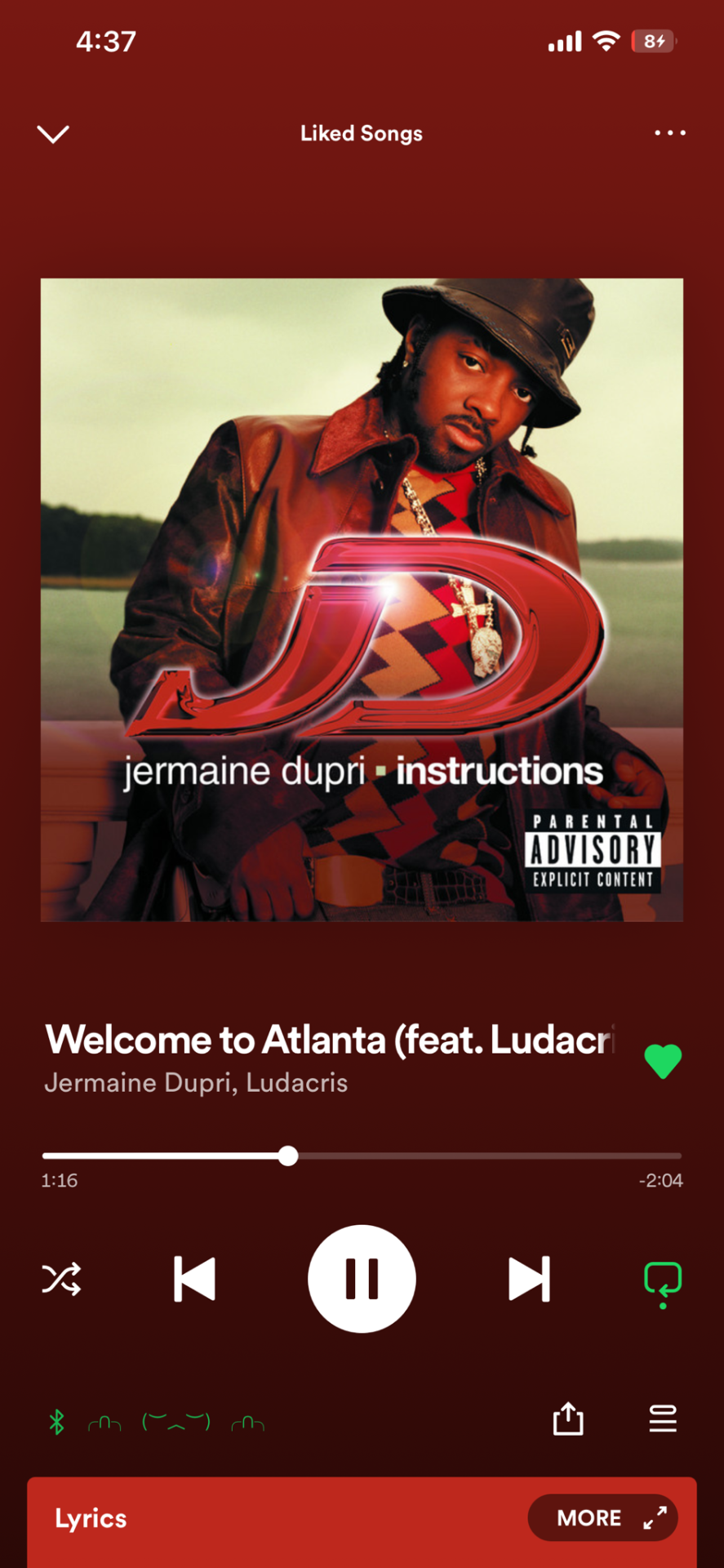The image shows a smartphone screen with a dark magenta background. The screen prominently displays a small square picture of Jermaine Dupri, who is wearing a suede jacket over a geometric print shirt and a hat. He is an African gentleman with a beard and mustache, and he has his head tilted slightly to the right, giving an inquiring look towards the camera. 

At the top of the screen, in white text, it shows the time "4:37" along with four bars indicating a full Wi-Fi signal. Next to the Wi-Fi icon, there's a status bar showing "8+" notifications. 

Below this, there's a down arrow followed by the text "Liked Songs..." indicating a navigation or dropdown menu. Beneath the picture of Jermaine Dupri, the text displays "Welcome to Atlanta (feat. Ludacris)", although "Ludacris" is abbreviated as "L-U-D-A-C-R."

A progress bar underneath indicates the current time elapsed in the song. Below the progress bar, there are control icons to skip to the previous track, play/pause, and skip to the next track. At the bottom of the screen, there are options for "Lyrics" and "More." Additionally, there's an icon to expand the screen display.

Overall, the screen interface combines various functional elements with the visual appeal of the artist, Jermaine Dupri.